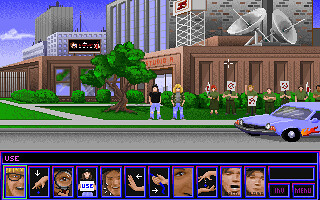The image appears to be a pixelated, 8-bit style screenshot from a video game, depicting a street scene in front of a brown brick building, possibly a radio or TV station, identifiable by two satellite dishes on its roof. In the center of the image stand two individuals on the sidewalk: one wearing a black shirt and blue jeans with dark hair, and the other with blonde hair wearing a grayish top and blue jeans. Additionally, there seems to be a couple of people holding picket signs, suggesting a protest. To the left of the main characters is a purple and reddish car with black wheels, and to the right, a blue vehicle. The scene includes a brown tree with green leaves, green grass, and a walkway. Various buildings are visible in the background, and the game's interface at the bottom of the screen includes character portraits and interactive icons like a magnifying glass, a hand, and the word "use," along with the abbreviations "INB" and "menu."